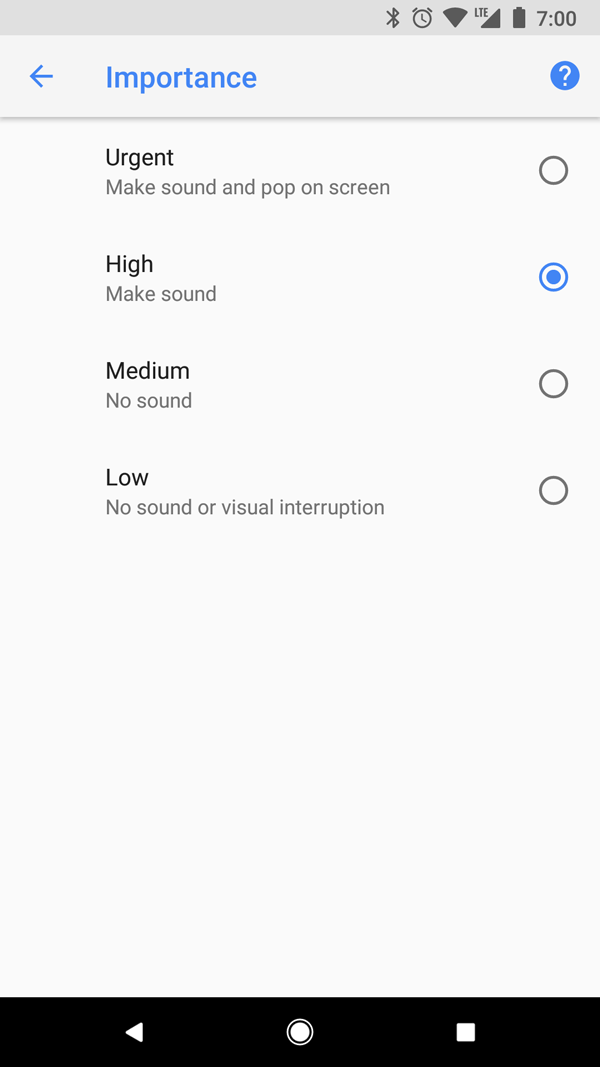A cropped screenshot of an "Alerts" tab within an app. At the top of the screen, the word "Importance" is displayed in dark blue font. To the left of this title, a back arrow icon allows the user to return to the settings page, while a question mark icon is situated on the right side for accessing additional information. Below, a vertical list of options categorizes alert notifications by their urgency level. These options include: "Urgent," "High (Make Sound)," "Medium (No Sound)," and "Low (No Sound or Visual Interruption)." The "Urgent" option is currently selected. The bottom of the screenshot features the black navigation bar of the phone, displaying the home button, the back button, and the square button to minimize the app. The background of the page is a neutral gray color, and the selected button is highlighted in blue.